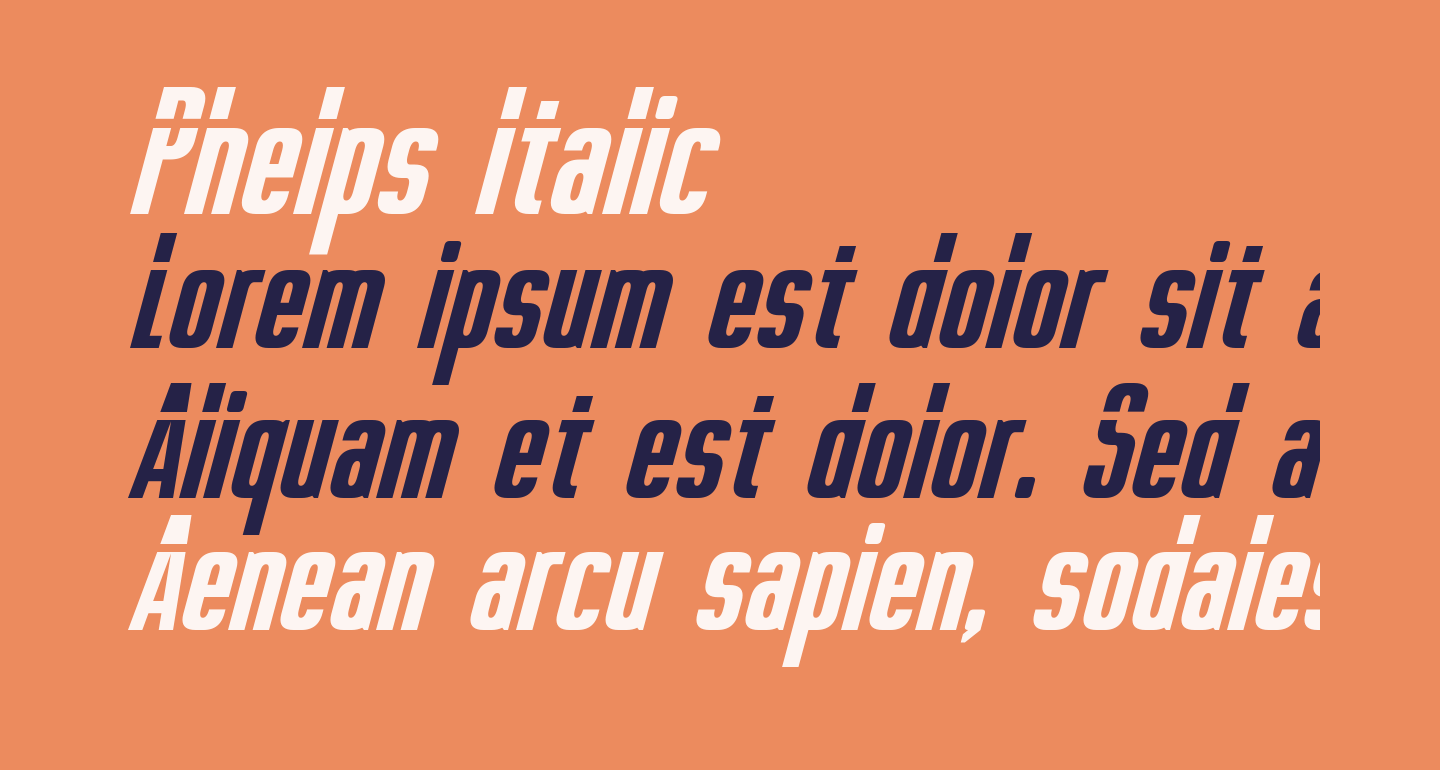The image features an orange rectangular background showcasing a font named Phelps Italic. The text is displayed in four lines. The first line, in white and italicized, reads "Phelps Italic," indicating the font name. The subsequent two lines, in dark blue, contain placeholder text resembling "Lorem ipsum," designed to demonstrate the font's style. Due to the font's distinctive characteristic, a negative space strip is carved out above the ascenders, truncating the tops of tall letters. The final line, also in white, contains more placeholder text, completing the sample display of Phelps Italic.